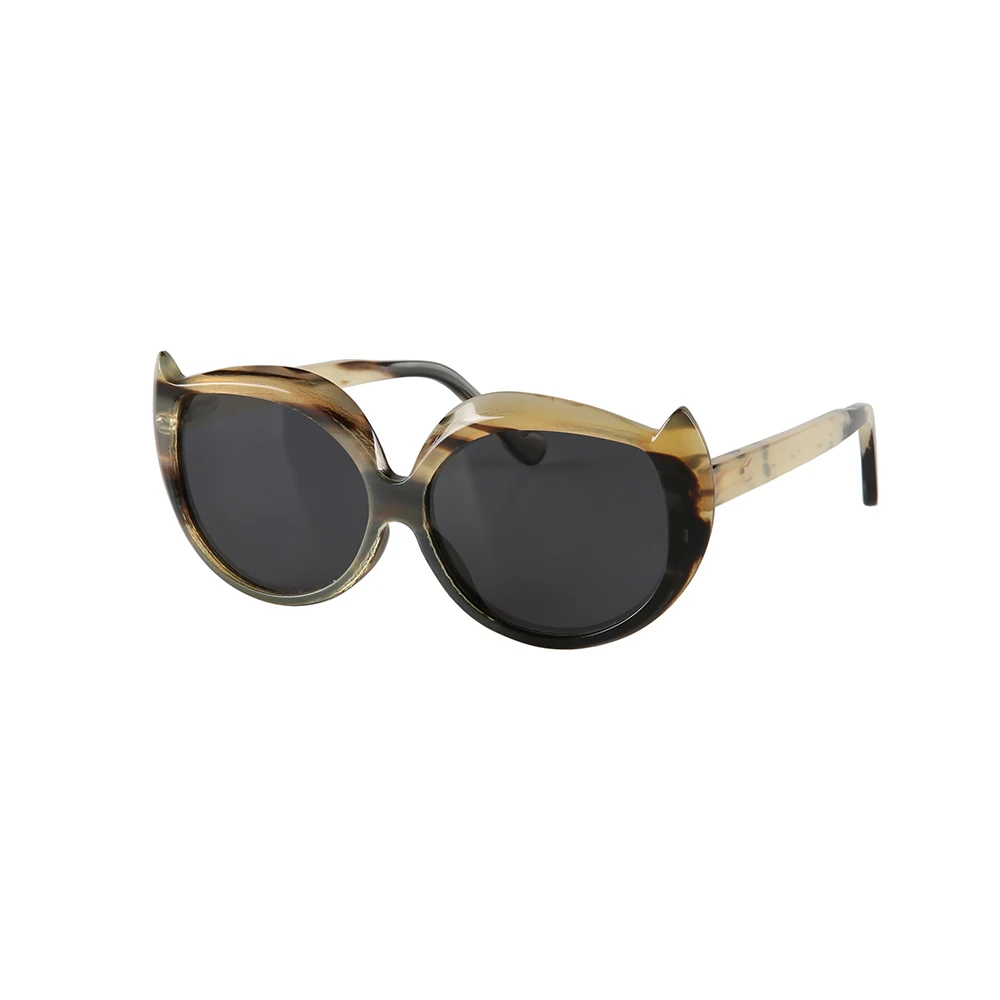The image depicts a pair of stylish sunglasses positioned at a slight angle to the left, with both the front and left side visible, as well as a glimpse of the inside right portion. The lenses are tinted dark gray, providing a stark contrast to the frame. The frame itself is predominantly light tan with variations in color throughout. The upper portions, especially at the top right and left corners, feature a mix of light tan and darker brown tones, giving a streaky turtle shell appearance. At the corners where the ear pieces meet the frame, there are distinctive, small protrusions resembling cat ears. The left lens’s edge and the upper part of the frame have darker streaks, while the inside portion of the right ear piece transitions from light to darker shades towards the back. Overall, the background is entirely white without any discernible surface or shadows, emphasizing the intricate details and color variations of the sunglasses. Notably, there appears to be some light-colored writing or markings on the outside of the left ear piece, though it is not legible.